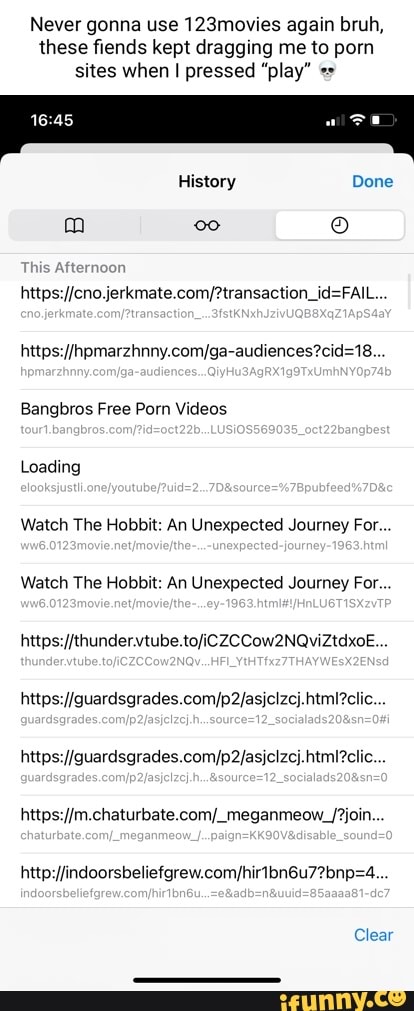The image features a book, a pair of glasses, and a clock, all highlighted against a stark white background. The setup conveys a sense of historical reflection, possibly alluding to the year 1645. Contrasting sharply with this serene and studious scene, there is a chaotic overlay of URLs and errant text referencing various dubious websites and pornographic content. This incongruous mix underscores the frustration of the narrator, who expresses disdain for ever using certain movie streaming sites again due to misleading links that direct to inappropriate sites.